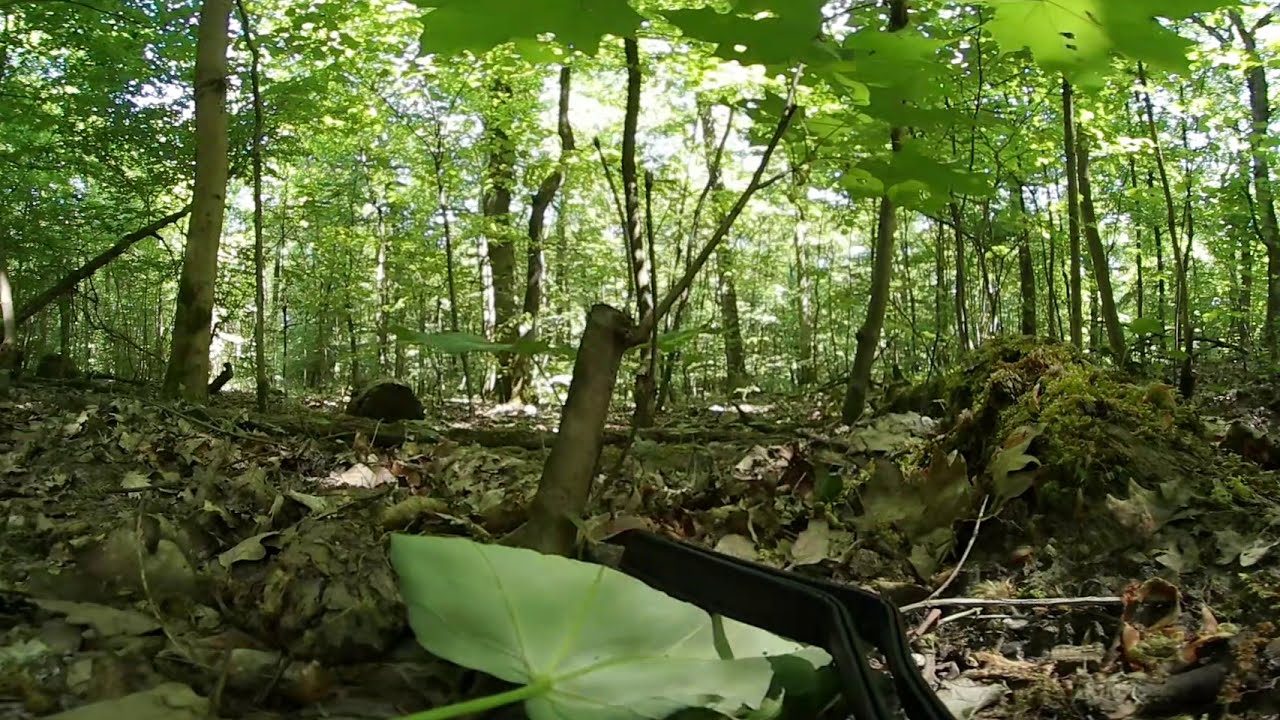This image was taken from a ground-level perspective in a dense forest, likely during the summertime. The forest floor is carpeted with a mix of light brown and reddish fallen leaves, interspersed with some green moss-covered logs. The scene captures a multitude of tall, thin trees with lush green foliage, indicating their relatively young age. The blue skies peek through the canopy, suggesting clear weather. In the bottom center of the image, a leaf appears to be slightly folded over, and a branch lies on the ground nearby. There is also a black object on the left side, possibly a camera strap, adding to the sense of the forest's natural setting. Additionally, the right side of the image features a moss-covered mound, further enriching the forest's verdant landscape.